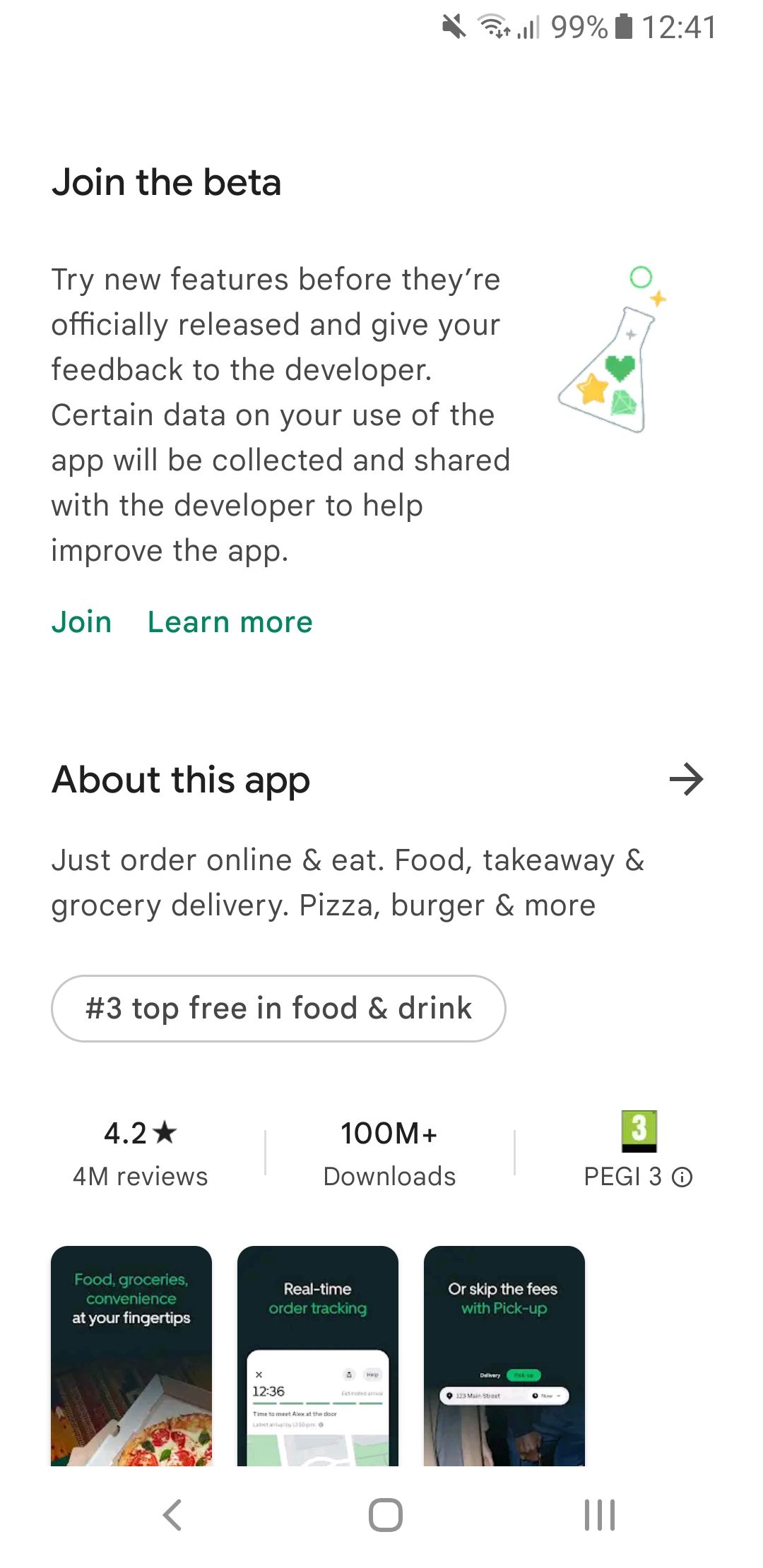Screenshot from a mobile device displaying detailed information about a food delivery app on Google Play or the Apple App Store:

At the top right of the screen, various phone icons are visible, including a mute button, Wi-Fi bars, data bars, a "99%" battery life icon, and the time displayed as "12:41". 

Below this, a section titled "Join the Beta" invites users to try new features before they are officially released and to provide feedback to the developer. It notes that certain data on app usage will be collected and shared to help improve the app. This section includes a clickable green button labeled "Join and Learn More." Accompanying this text is a small drawing of a beaker containing various symbols, including a green heart, a yellow star, and a green diamond.

Underneath, there is a header titled "About this App" followed by an arrow. The description below reads: "Just order online and eat. Food takeaway and grocery delivery, pizza, burger, and more."

A prominent label states the app's ranking as "Number 3 Top Free in Food and Drink." This is followed by a rating of "4.2" stars from "M" reviews, indicating the app has over "100M+" downloads. Additionally, there is a small label "PEGI 3" indicating the app's content rating.

At the bottom of the screenshot, there are three preview images showing highlights of the app.